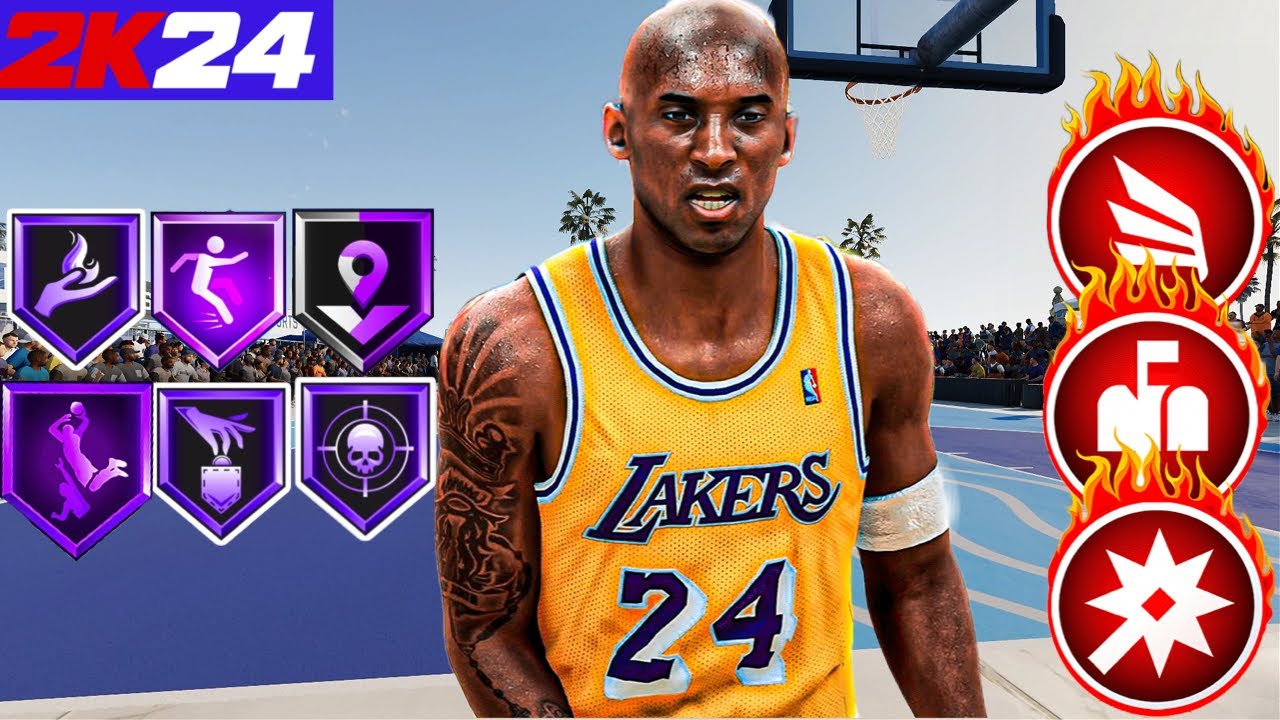This is a detailed and cleaned-up caption for the image described:

"A screenshot from the game NBA 2K24 showcases the interface. The top left corner displays the iconic '2K' logo in red, accompanied by '24' in white, signifying the latest edition of the series. Beneath the logo, a series of icons are neatly arranged, depicting various game features: a flaming hand, a high-jump symbol, a GPS marker, a crosshair with a skull, a gripping hand, and a player executing a dunk. Central to the screenshot is a prominent player wearing a yellow Lakers jersey, marked with the number 24. To the right, more icons are visible, including one resembling a mailbox and another shaped like a star at the bottom."